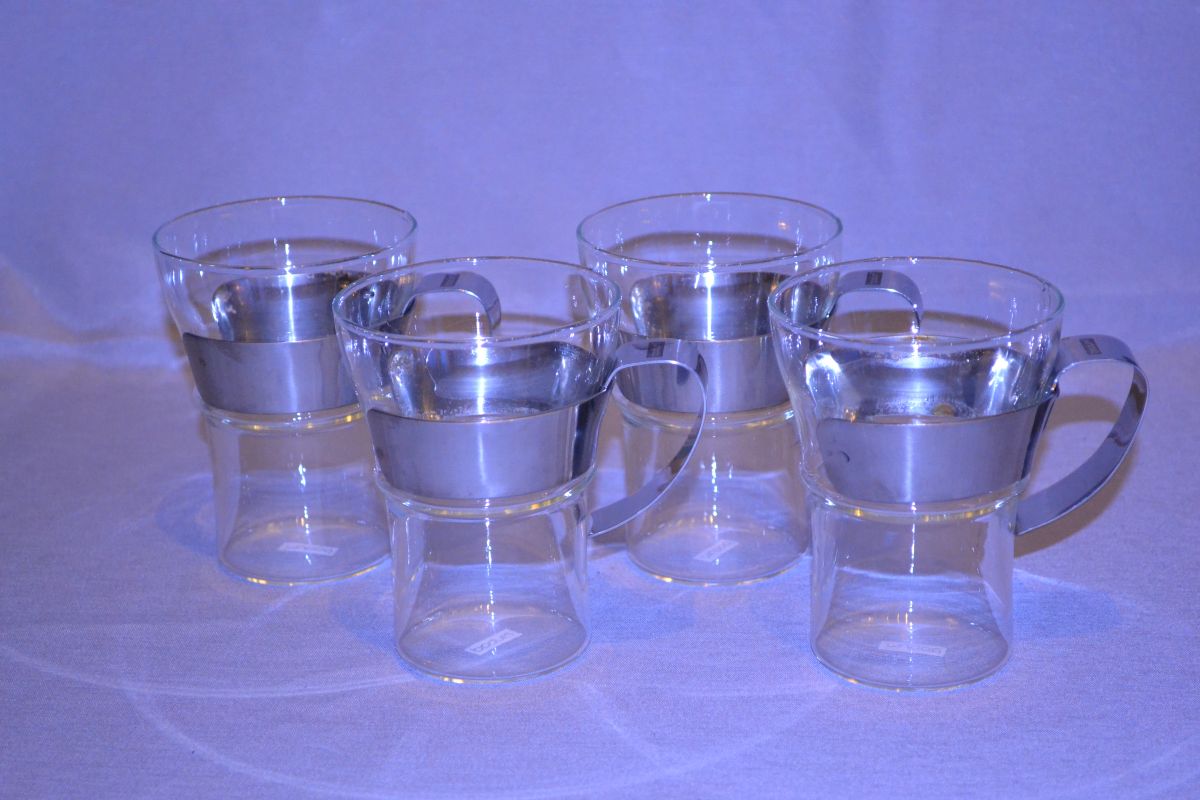The image features four identical clear glass mugs, each equipped with a distinctive chrome handle and a silver band encircling their midsection. These mugs exhibit a unique design where they are narrower at the bottom and widen towards the top. The glass mugs are neatly arranged on a light purple, almost violet, tablecloth that has subtle white marks, lending a glowing effect to the overall scene. Each mug has a small white rectangular tag at the bottom, likely indicating they are brand new. Despite initial uncertainty about their purpose, it appears they are tailored for drinks like tea or coffee and contain a clear liquid inside them. The background and surface seamlessly blend together, enhancing the aesthetic appeal of these elegantly designed mugs.